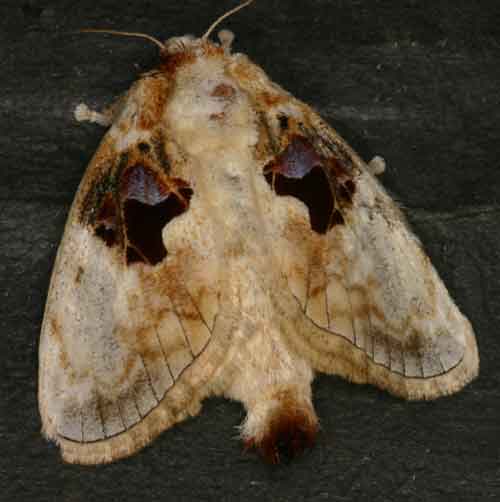This photograph presents an extreme close-up of a moth, filling most of the frame and appearing quite blurry due to the magnification. The moth, resting on what seems to be a dark, perhaps wooden surface, showcases its furry body and intricate wing patterns. The wings predominantly feature a light beige or off-white hue, interspersed with darker brown speckles and two prominent black splotches that resemble eyes or holes. These symmetrical splotches are located on the upper part of each wing, adding to the moth's distinctive appearance. The head, characterized by visible antennae, is positioned toward the top of the image, while the tail end faces closer to the bottom. Despite the blurriness, the moth's unique coloration and furry texture are clearly discernible, presenting a striking, almost stylized display.